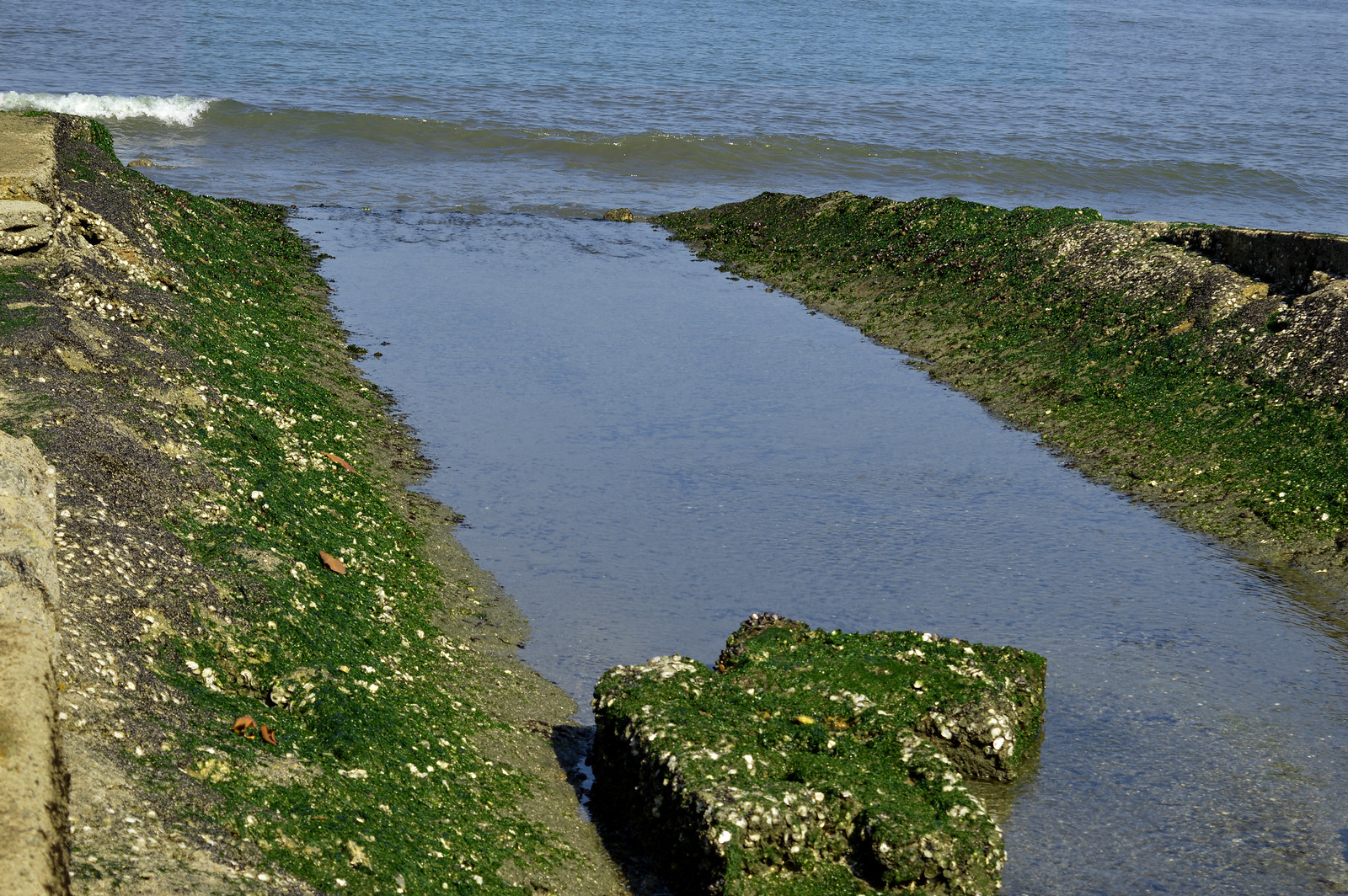The image captures a picturesque scene of a coastal environment, likely situated in a colder climate such as Iceland or England. In the background, a slightly wavy expanse of clear ocean or sea is visible, indicating windy conditions. A prominent wave is seen about to hit the rocky shoreline. The focal point of the image is a narrow inlet or stream of water extending inland from the larger body of water. This stream is shallow, only a few inches deep, and bordered on both sides by moss-covered rocks and jagged formations. Along the path of this water inlet, a large rock, also blanketed in green moss and seaweed, sits prominently in the middle. The edges of the stream are scattered with smaller rocks, grass, pebbles, and leaves, enhancing the natural and rugged beauty of the scene.